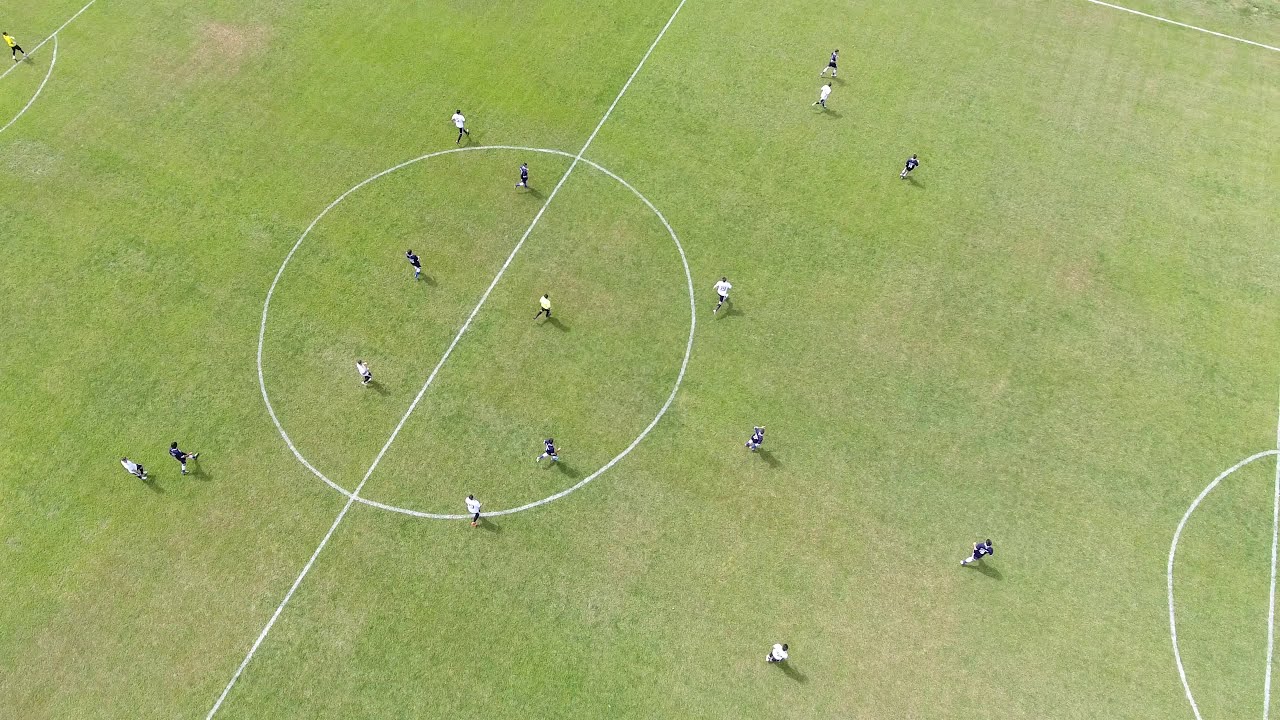This image captures a bird's eye view of an ongoing soccer match on a green field peppered with patches of brown dirt or dead grass. The field is marked with white lines, including a central line that runs diagonally from the bottom-left to the top-right of the frame, intersected by a white circle at its midpoint. Both goal areas are outlined, though the actual goals are not visible in the photograph. Scattered across the field are 16 tiny figures, resembling ants from this high vantage point, all in motion with their legs akimbo, heading in the same direction. The players are distinguished by their uniforms: one team in dark blue jerseys, the other in white. Additionally, a goalie in a neon yellow jersey is positioned in the top-left corner. Shadows are visible beneath the players, adding depth to the scene.